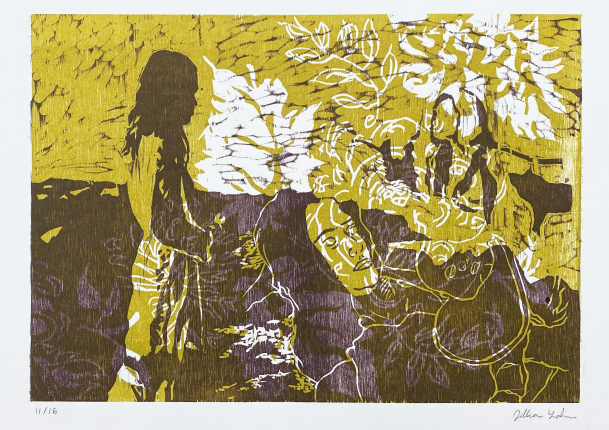This detailed artwork features a rectangular composition with a distinct gray border, accentuating the vibrant and surreal inner scene. Predominantly hued in shades of yellow, black, gold, and white, the painting captures a blend of ethereal and grounded elements.

At the top of the artwork, a yellowish sky merges with white, leaf-like areas indicative of trees, creating a serene yet abstract backdrop. The bottom half transitions into darker hues of black and dark purple, suggesting a shadowy ground interspersed with white patches resembling leaves and plants.

Central to the artwork are three human figures. To the left, a woman stands prominently. Clad in yellow, her face and arms are rendered in solid black, without intricate details, emphasizing the figure's silhouette through shading. On the right, partially blending into the yellow background, another woman is depicted in a sitting posture. Additionally, there’s a distinctive yellow face, partially obscured, looking rightwards from the middle of the image, adorned with long black hair.

The figures' attire suggests influences from Hindu or New Age Transcendentalist cultures, adding an element of mysticism to the scene. The artist's signature is placed on the bottom right corner in cursive, though it remains illegible due to its small size. The numbers "11-16" can also be seen on the bottom left of the composition.

This complex interplay of colors, forms, and cultural references makes for an intriguing piece that invites speculation and deeper analysis.